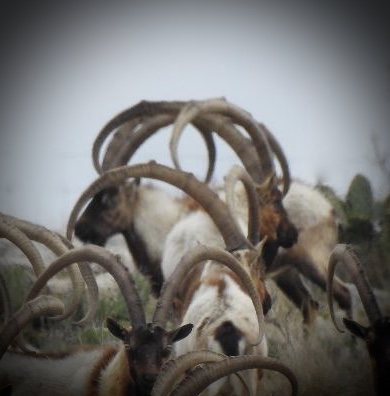In this slightly blurry, outdoor photograph, a group of majestic antelope, possibly ibexes or long-horned sheep, are captured in a natural, rugged setting. The image, characterized by a special lens effect, creates a soft, out-of-focus ambiance, particularly around the edges and corners, with a distinct white haze or halo above the animals. The antelope have striking, very long, curved horns that appear dark brown or gray, so extensive that they almost obscure their bodies, creating an intricate spectacle of interwoven horns. The animals, clustered together in tall grasses and rough vegetation, display a mix of coloration: dark brown or black heads, whitish bodies with reddish-brown and brown spots. A gray, overcast sky forms the backdrop, contributing to the overall muted and ethereal atmosphere of the scene.